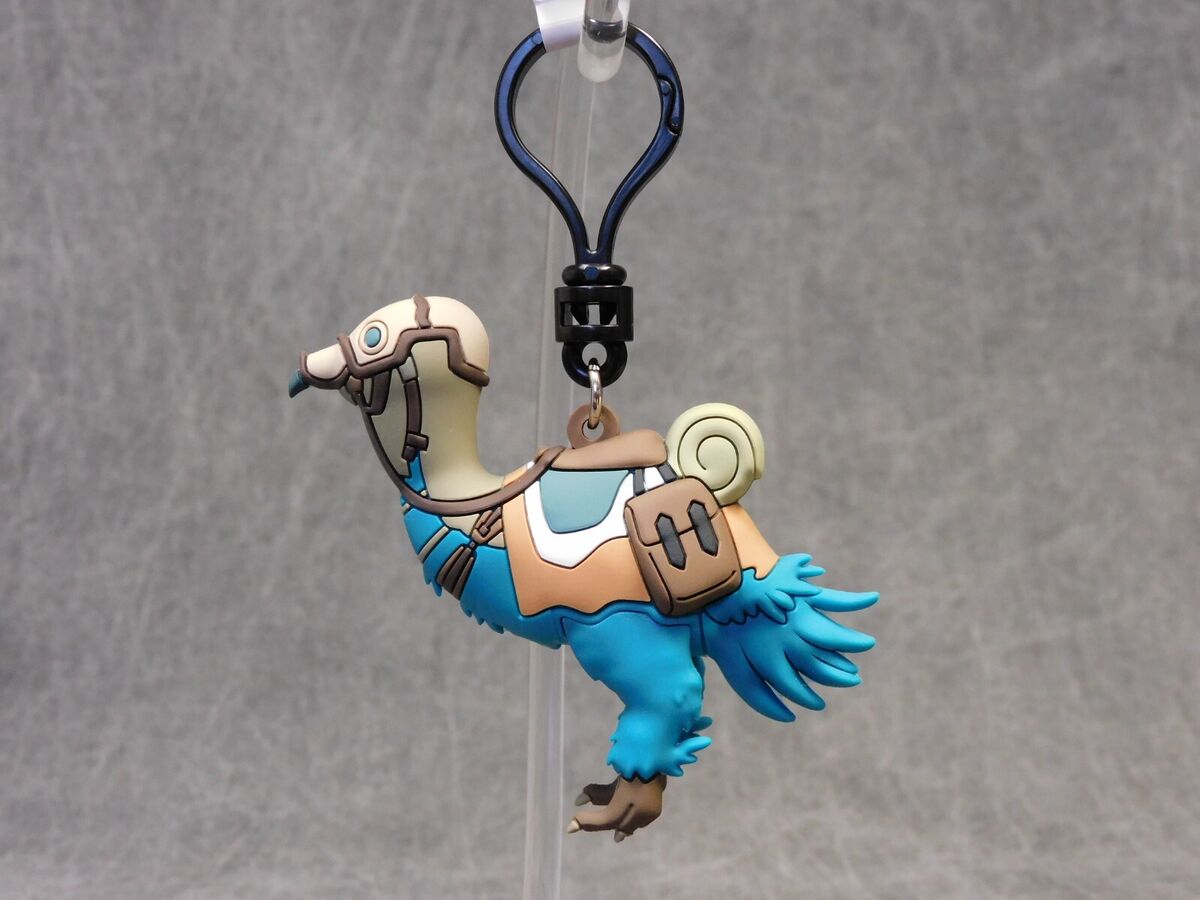The photograph features a fantasy blue bird, possibly serving as a keychain or Christmas ornament, hanging from a fully enclosed metal hook. The bird, resembling an ostrich or turkey, is adorned with a harness and saddle, giving it the appearance of a creature meant for riding. The saddle is blue and detailed with brown elements, including a brown sack affixed to it. Between the saddle and the bird's body, there appears to be a blanket or padding, and a rolled-up sleeping bag is positioned at the back of the bird. The bird’s head and neck are covered by a pale, leather-like helmet with straps, resembling old-time aviator gear, though it lacks goggles. The bird's beak peeks out from under this head covering, adding to its whimsical, fantasy appearance.